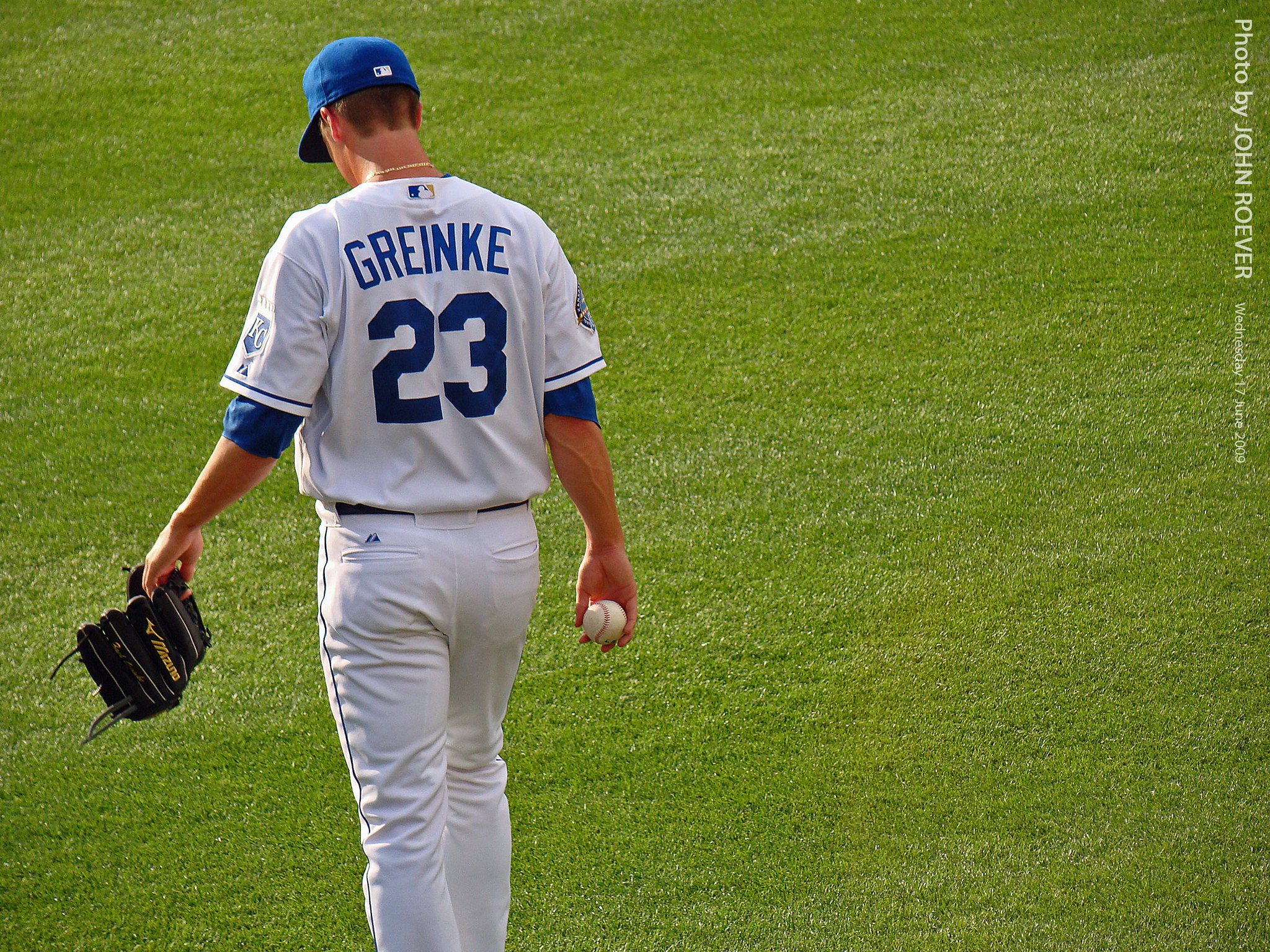This is a dramatic photograph of a baseball player walking away on a perfectly manicured field, captured in a slight landscape view, close to square. The player, centrally positioned in the center left of the image, is shown from behind, slightly below the calf upwards. He is wearing a white uniform with blue accents: a blue cap, a blue long-sleeve shirt under his jersey, and white pants with blue stripes down the sides. His jersey prominently displays the name "Greinke" and the number "23" in large blue text across the back. He holds a baseball in his right hand and a black glove with a yellow logo and text in his left, held upside down. A gold chain peeks out from under his jersey. The entirety of the background is filled with lush green grass. Additionally, there's a small text in the upper right corner that states, "Photo by John Rover Wednesday 17 June 2009."